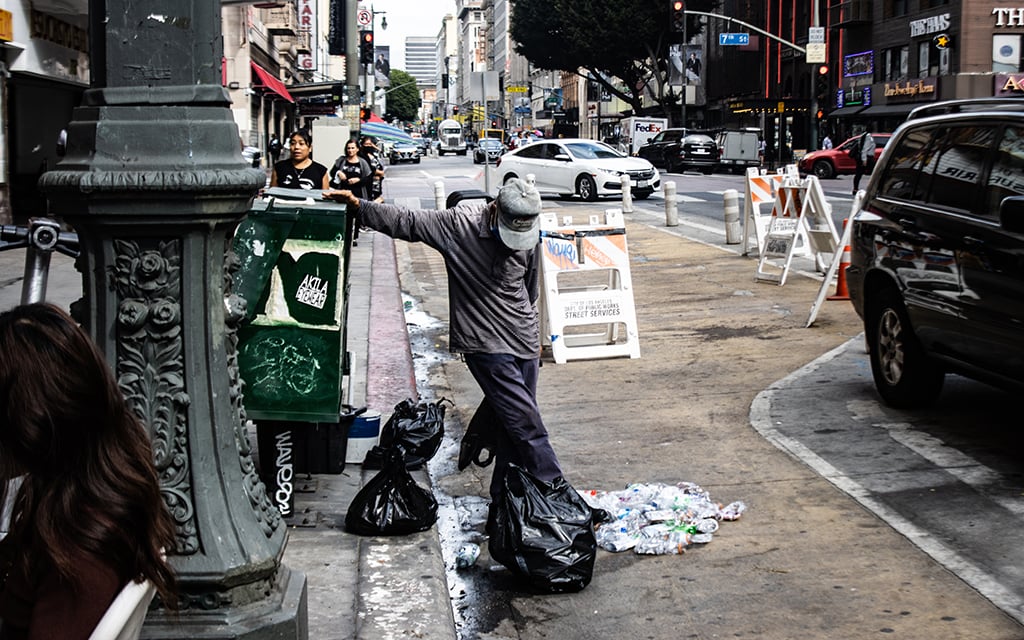This detailed, realistic black-and-white photograph captures a busy urban street scene, presumably in Manhattan, New York City. Central to the image is a man dressed in grey clothes and a cap, who is leaning on a green, possibly a mailbox or garbage can, while looking down at the ground where heaps of black trash bags—some spilling out their contents—are scattered around his feet. His right hand stabilizes him against the green item, and his legs are crossed, right over left. Behind him, a series of white and orange construction barricades line the street, which is bustling with activity.

The background features a variety of vehicles, including a black SUV parked to the man’s left, a white car moving not entirely on the proper lane, a pickup truck, and a recognizable FedEx truck, suggesting a typical busy day in the city. There are also notable street elements like a green light pole on the left side and a sign potentially indicating "7th Street" hanging from a lamppost.

Pedestrians walk along the sidewalk, which appears dirty with occasional spilled trash, while glimpse of city life happens with someone sitting on a bench and others mingling in the background. The photograph offers various shades of grey, emphasizing the contrasts and textures of the urban environment, from the streetlights to construction motifs, creating a chaotic yet familiar city atmosphere.